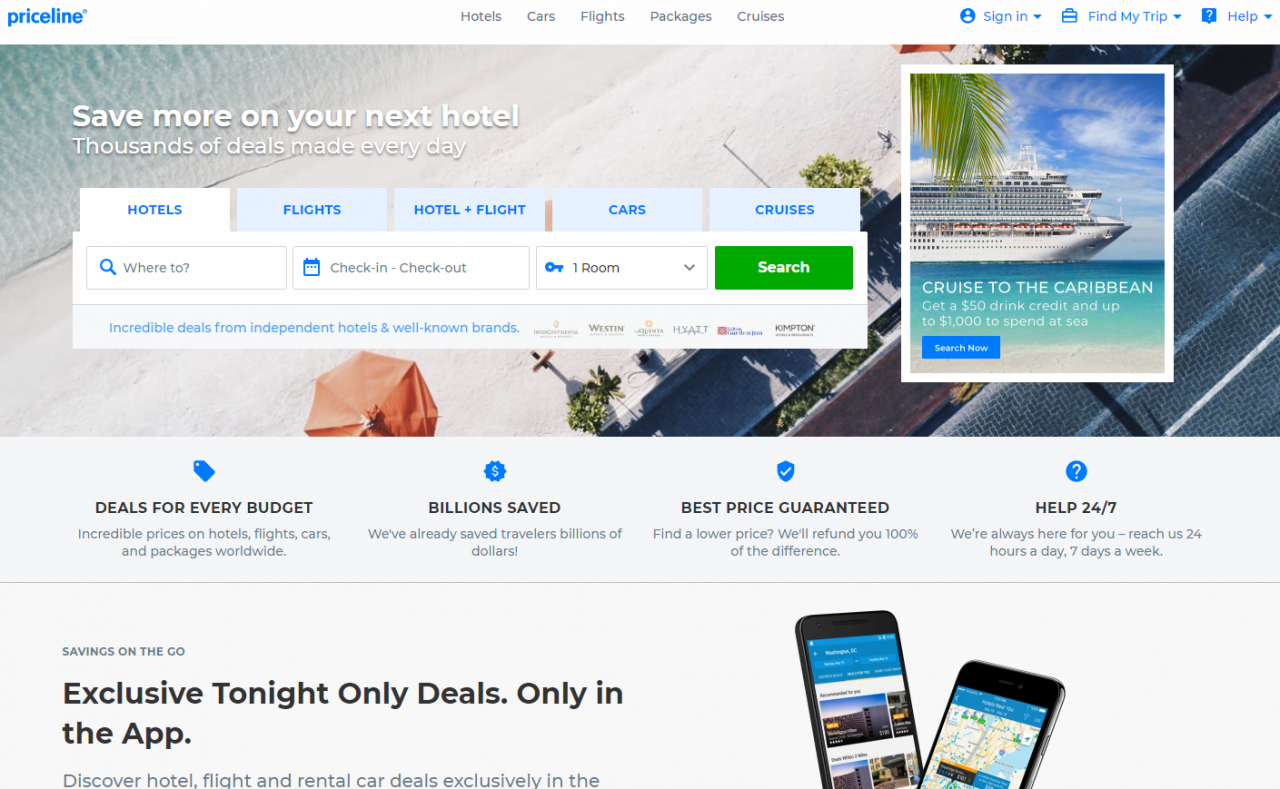The image depicts a website interface for Priceline. In the top left corner, the "priceline" logo is displayed in blue lowercase font. The logo is positioned on the left side of a horizontal menu bar. Centrally located on this menu bar are the main navigation options: "Hotels," "Cars," "Flights," "Packages," and "Cruises." Aligned to the right are additional options such as "Sign In," "Find My Trip," and "Help."

Beneath the menu bar is a banner featuring an aerial shot of a beach, inclusive of a house, an umbrella, and what appears to be either a roadway or the top of a roof, partially emerging from the bottom right corner of the image. The banner's textual overlay promotes savings with the message: "Save more on your next hotel. Thousands of deals made every day."

Directly below the banner are tab options: "Hotels," "Flights," "Hotel + Flight," "Cars," and "Cruises." These tabs sit above a search bar where users can input their travel details such as destination, dates, and number of rooms.